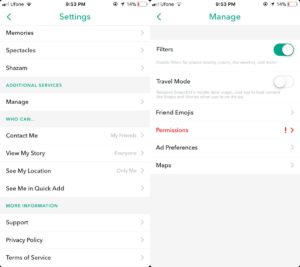The image consists of two side-by-side cell phone screenshots. The screenshot on the left is labeled "Settings" and contains four distinct sections. The top section is labeled "Memories," but the text beneath it is somewhat blurry and appears to mention "Shazam." Following this, there is a section titled "Additional Services."

The screenshot on the right is labeled "Manage" and has three sections. At the top of this screenshot, notifications display the current time and a cell phone icon, mirroring those seen on the "Settings" screenshot. In the "Manage" section, the first option is "Contact Me," followed by "View My Story," "See My Location," and "See Me in Quick Add."

Underneath these, there are additional options: "Filters," which is toggled on, and "Travel Mode," which is toggled off. The final options mentioned are "Friend Emojis" and "Maps."